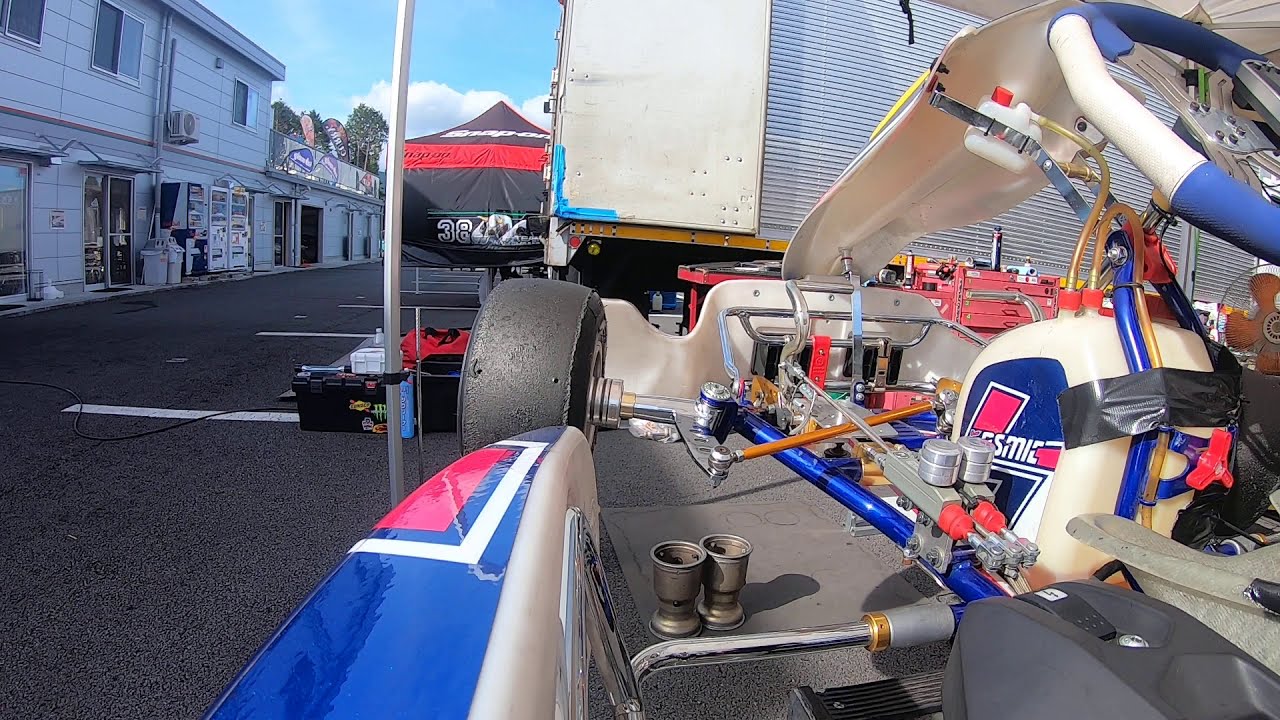This detailed close-up image showcases a Formula One-style racing car that appears to be undergoing maintenance. Central to the image is the car itself, which prominently features a variety of colors including reds, blues, whites, blacks, golds, and grays. The car, with text possibly reading "SSMIC" on it, shows intricate details such as the steering wheel, the seat, and parts of the engine or gas tank, emphasizing the mechanical components typical of an F1 vehicle. Positioned from a perspective that places the viewer within or very near the car, the front end is highly visible and set slightly to the right.

In the background, several elements add context to the scene. Directly above and to the right of the car is the back of what seems to be an 18-wheeler, colored in gray, white, and yellow. To the left of this is a red, black, and white awning that has the text "SNAP-ON" and the number "38," possibly indicating a tent associated with a radio station advertisement featuring a singer with a microphone. Further to the left, the black concrete road with white lines extends, leading to a gray-colored building on the far left, which includes what looks like three garage stalls.

The overall setting suggests a busy pit stop or garage area with clear skies, where the car is being prepared, potentially for an imminent race, highlighting the prepping process through the visible wheel bearings and the worn tires awaiting repair. The detailed and vibrant depiction captures the crucial stages of race car maintenance amidst a backdrop of related racing infrastructure.